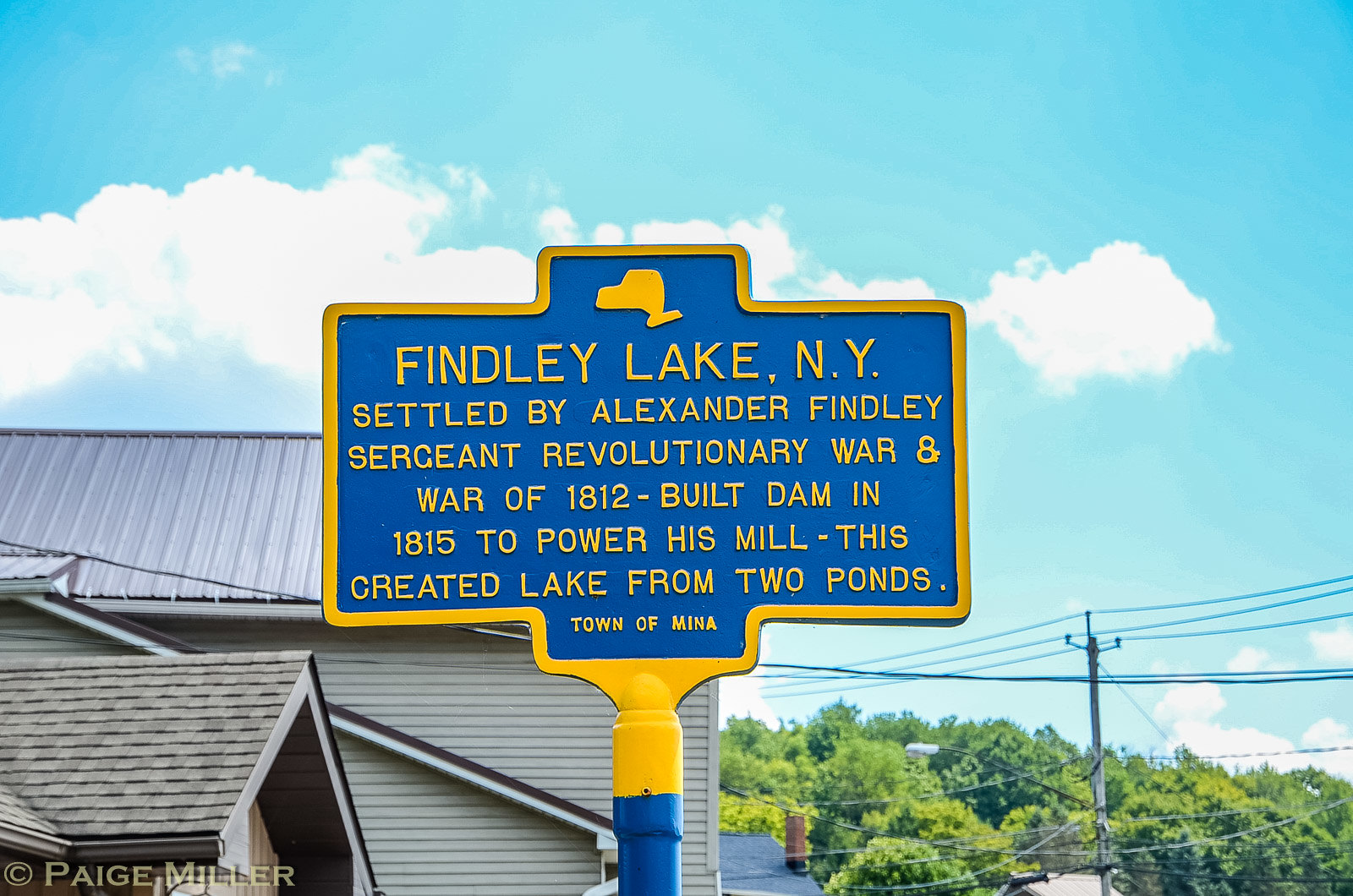The photograph, a horizontal rectangular image, features a prominently positioned sign in the center. This sign, mounted on a blue pole, exhibits a dark blue background with a light yellow border and header resembling the shape of New York State, akin to the Chevrolet logo. The inscription on the sign, all in capital letters with varying sizes, conveys the historical significance of Finley Lake, New York: "Settled by Alexander Finley, Sergeant Revolutionary War and War of 1812. Built dam in 1815 to power his mill. This created lake from two ponds. Town of Mina." Surrounding the sign, the setting is idyllic with a combination of residential buildings, trees, and power lines seen towards the bottom right. The backdrop reveals a bright blue sky with some clouds, indicating it is a clear, sunny day in what seems to be a quaint small town. The buildings feature shingle roofs and siding, contributing to the picturesque, small-town atmosphere. Additionally, various colors are present in the image, including light blue, white, gray, yellow, dark blue, brown, and different shades of green.